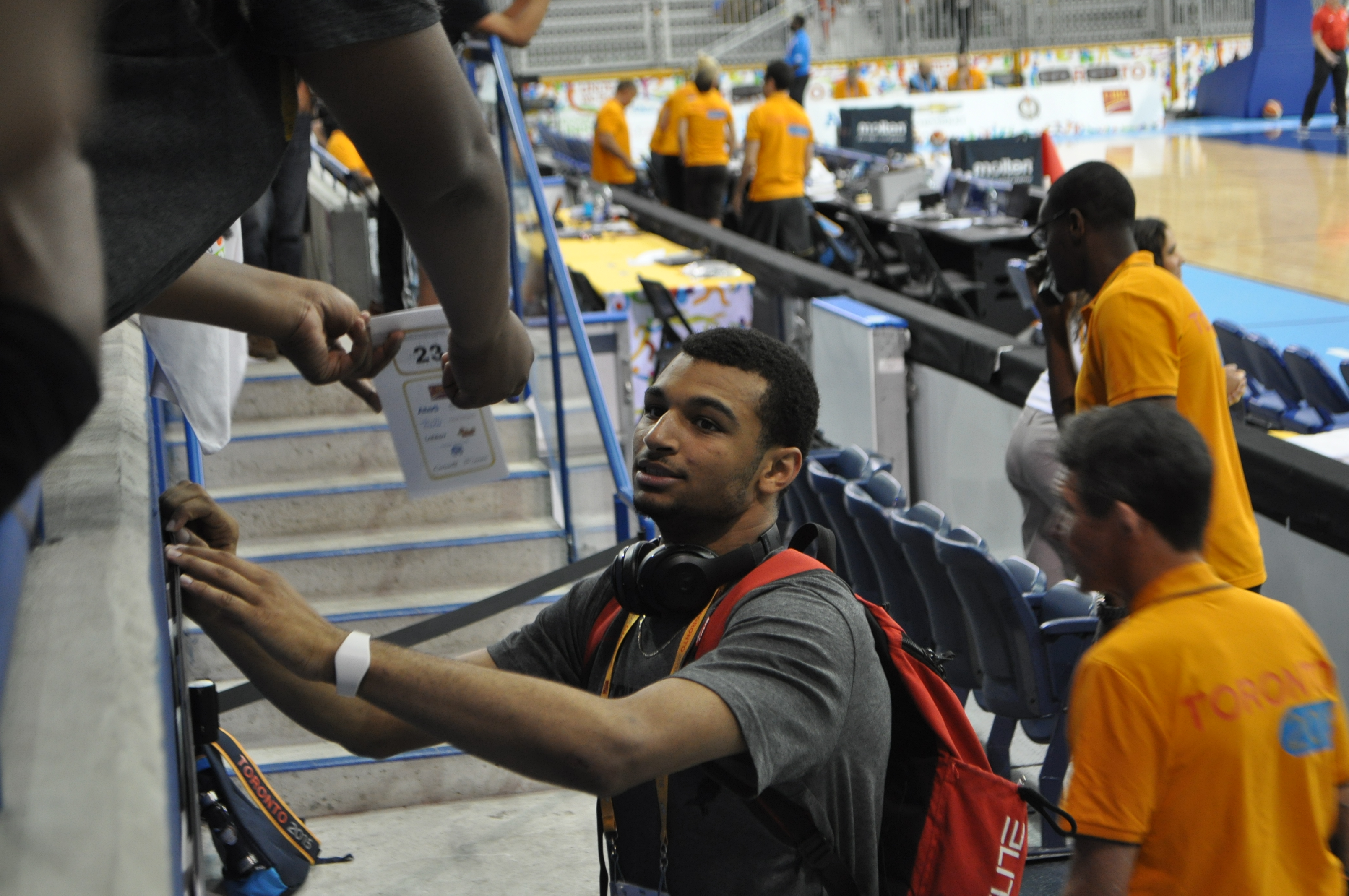In this detailed color photograph taken in an indoor basketball court, the main focus is a man standing at the bottom of an audience seating area on a concrete walkway. He has very short hair and is dressed in a gray short-sleeved t-shirt with a thin gold chain around his neck. He is partially facing away from the camera, with a red backpack with white lettering on it strapped over his shoulders. Around his neck, he wears black over-the-ear wireless headphones, and on his arm, there's a white wristband. His hands appear to be engaged in an activity near a concrete wall, where someone is leaning over from above, holding a white piece of paper with the number 23 in black and orange outlines, presumably seeking an autograph.

To the man's surroundings, the basketball court with its polished wood flooring and various blue marked play areas is visible in the background. At the top right of the image, there's a person dressed in black pants, white shoes, and a red polo shirt. Looming in the far background is a table covered with a white tablecloth with several black seats behind it, occupied by multiple people.

Scattered around the man are several other individuals, many of them wearing orange shirts with red writing that says "Toronto" and bearing a blue emblem. There are at least six identifiable men in orange shirts: four at the top and two directly behind him. A blue guardrail runs up some stairs on the left of the image, indicating the audience seating area. The scene gives the impression of a post-game moment, possibly involving fans seeking autographs from the player.